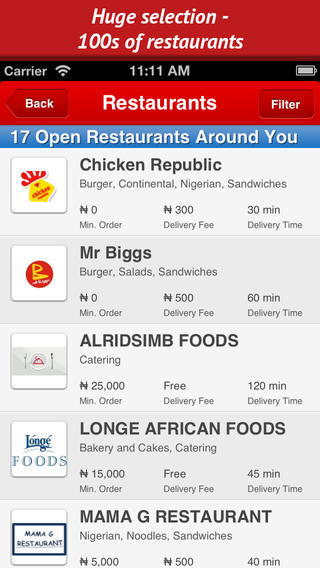The screenshot displayed on the screen showcases a food delivery application interface with a vibrant mix of colors and detailed information. At the top, the status bar indicates it's 11:11 AM, the device has a full battery, and it's connected to a wifi network. Just below, in a bold red label with white text, the word "Restaurants" is prominently displayed. To the left of this label, there is a back button, and to the right, a filter option for refining search results.

In the middle of a blue background, white text announces "17 open restaurants around you." The list of restaurants starts with "Chicken Republic," which offers burgers, continental cuisine, Nigerian dishes, and sandwiches. There's no minimum order fee, the delivery charge is 300, and the estimated delivery time is 30 minutes.

The second restaurant, "Mr. Biggs," features burgers, salads, and sandwiches. Again, there's no minimum order, but the delivery fee is set at 500, with a longer delivery time of 60 minutes.

"Allrids Foods" comes next, specializing in catering services. Here, the minimum order is quite substantial at 25,000, though delivery is free. The delivery time is notably longer, estimated at 120 minutes.

Following that, "Loaned African Foods" offers bakery and cakes, as well as catering services. The minimum order is 15,000, delivery is free, and the estimated delivery time is 45 minutes.

Lastly, "Mama G Restaurant" rounds out the list with Nigerian dishes, noodles, and sandwiches. The minimum order is 5,000, with a delivery fee of 500, and the estimated delivery time is 40 minutes.

The overall background of the app is predominantly white, featuring restaurant logos and text in black, enhancing readability.